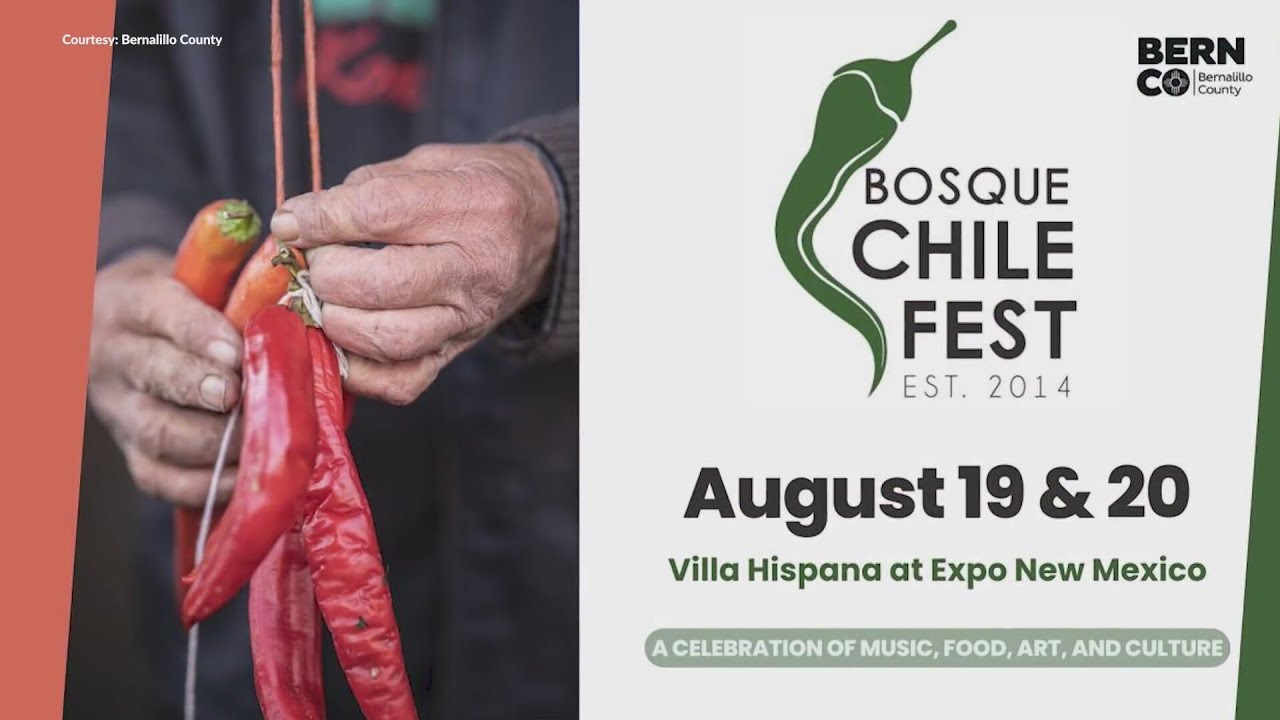This advertisement for the Bosque Chili Fest prominently features a photograph on the left half of an elderly man's wrinkled hands holding a bushel of vibrant peppers. The man's black t-shirt, adorned with red text, and his dark grey or black jacket form the background, which is artfully blurred to emphasize the peppers in his grasp. The peppers themselves are long and thin, vividly red at the front, with two smaller orange-topped peppers nestled in his hands.

The right half of the ad features a clean white background with a series of typographic elements and logos. At the center is a green pepper-shaped logo, flanked to the right by text that reads "Bosque Chili Fest" in black, with "EST. 2014" noted below in a thinner font. The top right corner contains a logo comprising the text "BERN," an ornate "C.O," and the phrase "Bernoullio County" in smaller text beside a thin vertical line.

Prominently displayed in bold block text on the lower portion are the event dates, "August 19 & 20," followed by "Villa Hispana at Expo New Mexico" in green text. At the bottom of the white panel, a horizontal pale green oval houses the phrase "a celebration of music, food, art, and culture" in white text. The advertisement is watermarked in the top-left corner with the text "courtesy Bernoullio County." This visually cohesive design effectively communicates the festive atmosphere and cultural celebration of the event.